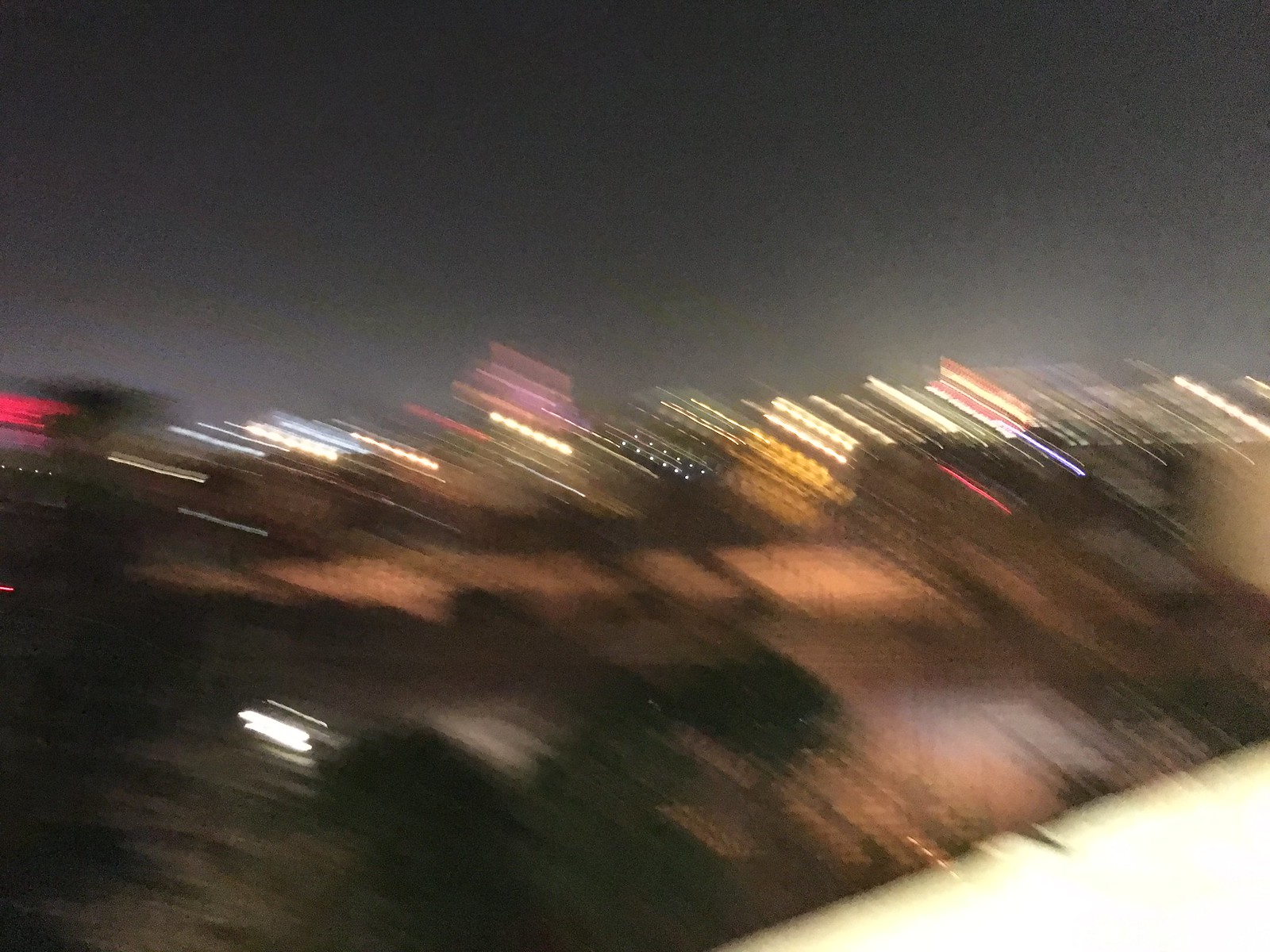A nighttime outdoor scene captured in a completely blurred and distorted photograph. The sky at the top of the image merges in hues of black and gray, creating a moody backdrop. Short, streaking lines suggest the presence of distant lights and faintly discernible buildings on the horizon, where city lights subtly illuminate the sky. The bottom left corner of the photo plunges into deep darkness, in stark contrast to the bottom right corner, which is overwhelmingly bright and washed out, forming a bright angle that dominates that part of the image. The overall impression is one of a cityscape swallowed in ambiguity and motion.